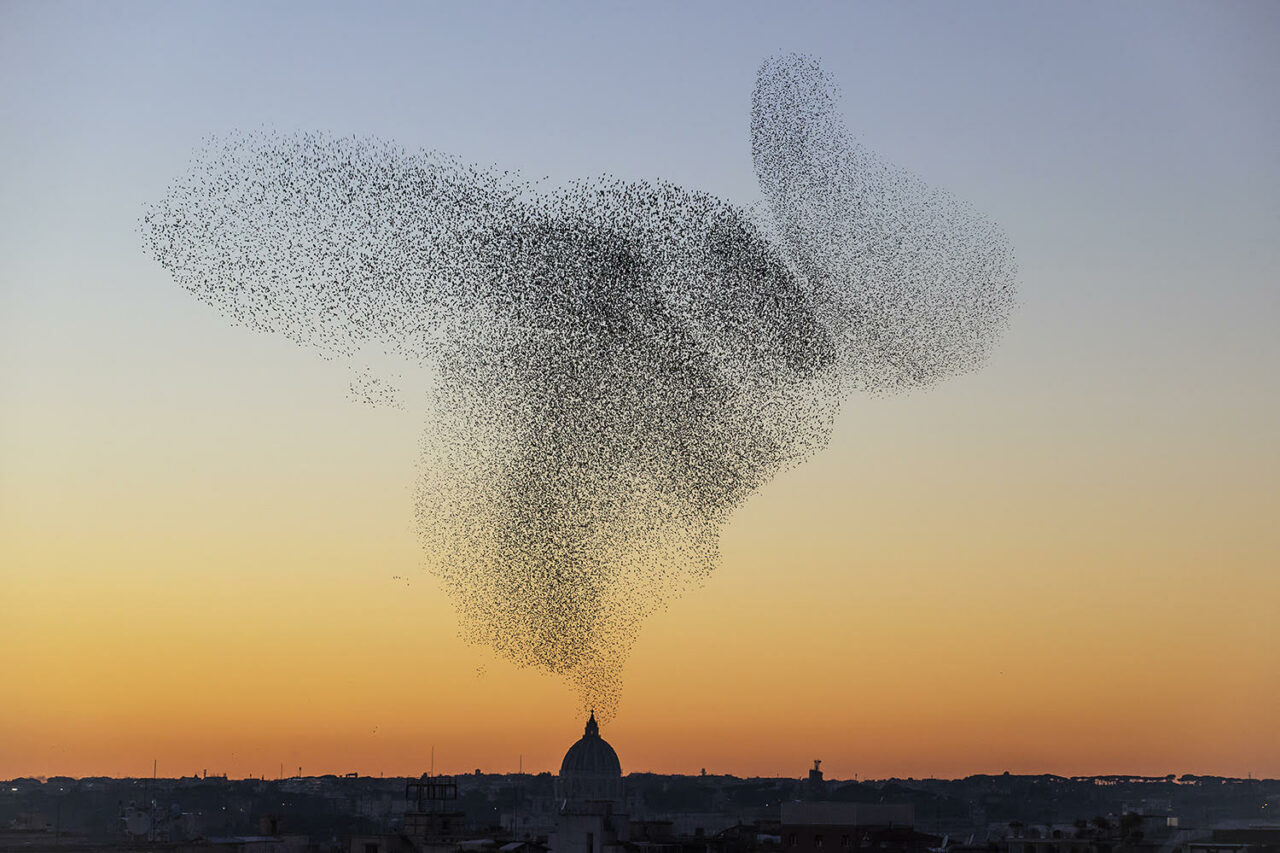The photograph captures a mesmerizing cityscape at either dawn or dusk. The sky features a stunning gradient, transitioning from a medium dark blue at the top to darker blues and hints of grey before blending into vibrant gold near the horizon, with a final touch of dark gold right where the land meets the sky. The city below is characterized by multiple domed buildings, suggesting a possible Middle Eastern location, reminiscent of mosques.

A particularly notable structure is a taller, domed building that stands out among the others. The true fascination, however, lies above this domed building, where a massive cloud of swirling birds—numbering in the millions—create an aerial spectacle. This swarm forms intricate patterns in the sky, which some might even liken to familiar shapes, such as the face of Snoopy, the beloved cartoon dog from the Peanuts series. The overall scene is bathed in the ethereal light of a transitioning sky, making the natural and urban elements blend seamlessly in this captivating image.